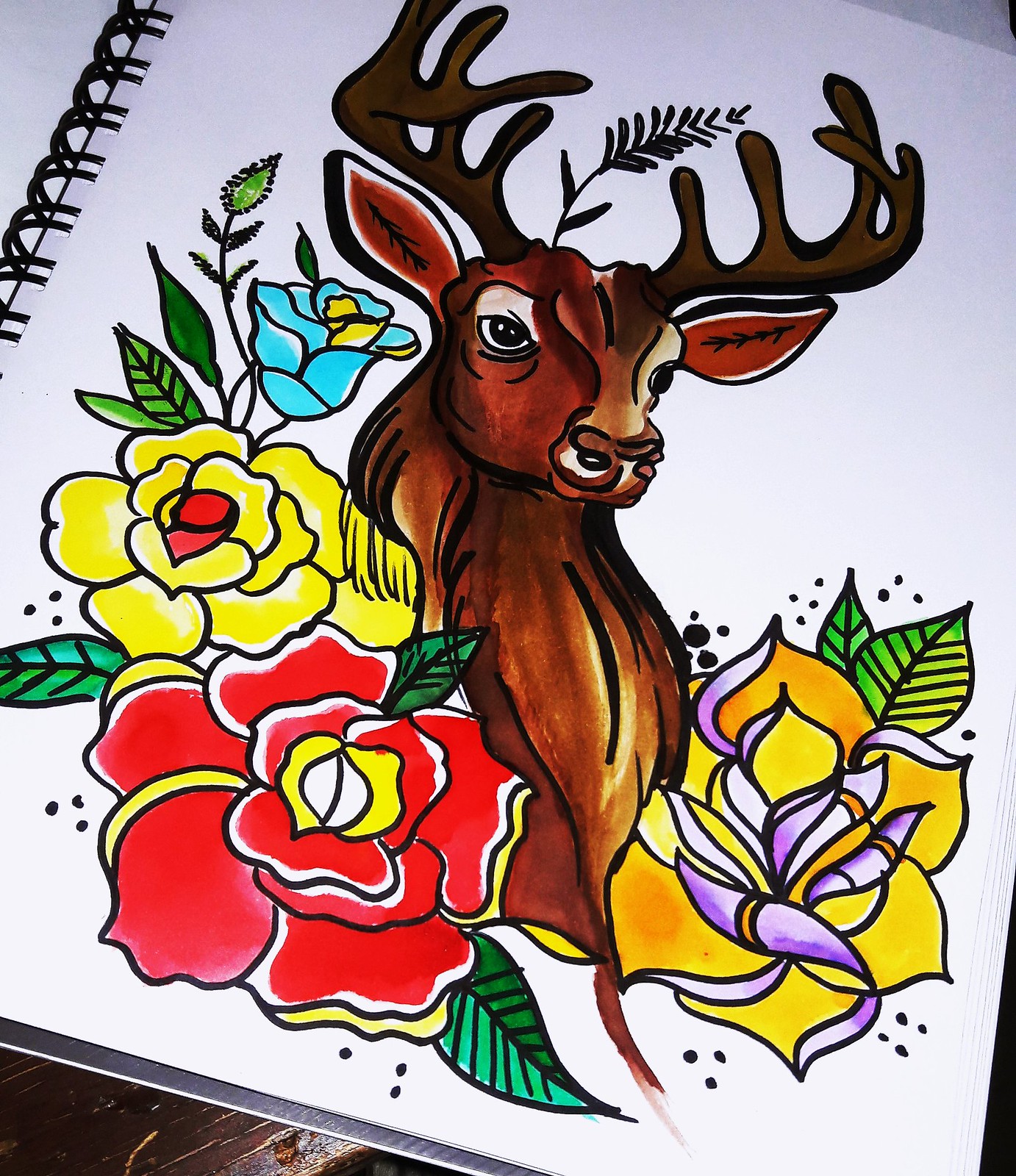This is an artistic drawing rendered with markers, depicting a majestic brown moose at the center of the notebook page. The moose is oriented such that its head is slightly turned, gazing towards the center right of the image. The surrounding scene is a vibrant array of flora, with noticeable yellow, red, and purple flowers encircling the moose. Adding to the eclectic composition, a fern extends upwards from the moose's head, enhancing its majestic appearance. The background of the image subtly reveals the spine of the notebook in the top left corner, grounding the focal illustration within the context of the notebook page. The overall look of the drawing gives an impression of being AI-generated due to its distinct style and vivid details.